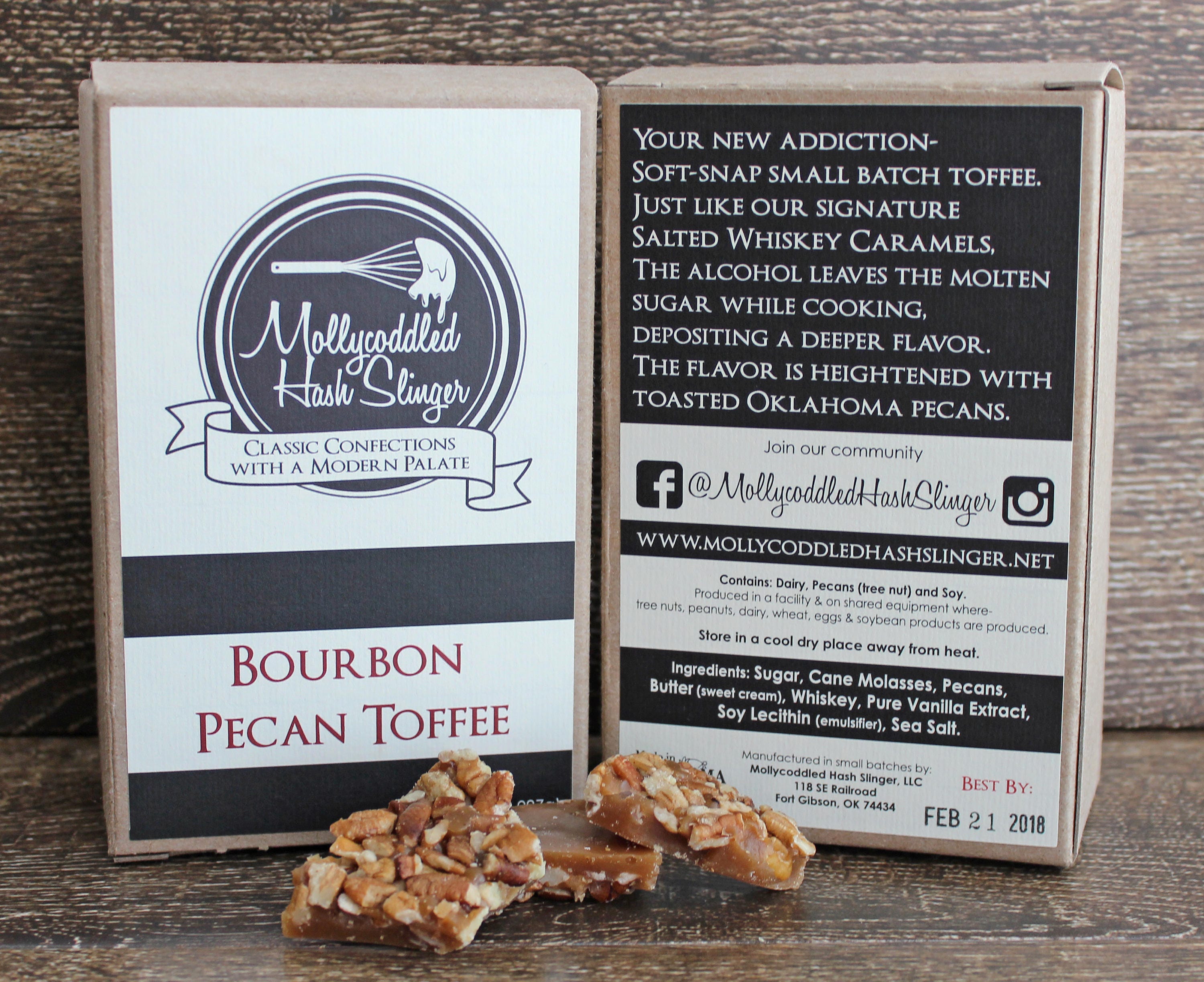The image depicts two elegant black-and-white boxes of Bourbon Pecan Toffee from Molly Coddled Hash Slinger, a brand known for its classic confections with a modern palette. The box on the left showcases the front, which features the brand's name and product description, emphasizing the formal and classy design. The box on the right reveals the back, detailing the toffee as a small-batch product with a soft snap, similar to their signature salted whiskey caramels. The description highlights the unique preparation process where alcohol leaves the molten sugar during cooking, enriching the flavor which is further enhanced by toasted Oklahoma pecans. Visible on a wooden backdrop, three toffee pieces lie between the boxes, showcasing the product. Additional details include a best-by date of February 21, 2018, and links to the brand’s community and social media at www.MollyCoddledHashSlinger.net.